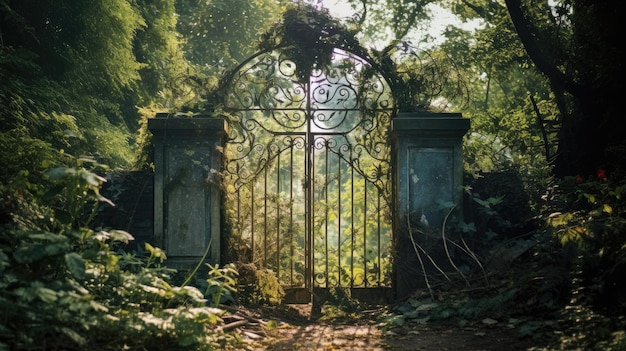This photograph captures an old, ornate wrought iron gate with a thick patina of age, standing as the focal point against a verdant backdrop. The gate, with its intricate flourishes and overgrown vines wrapped around its arch, is framed by two imposing stone pillars. Each pillar reaches almost to the top of the gate and has branches and other vegetation leaning against them. Extending from these pillars are walls, largely concealed by the lush greenery surrounding them. Tall trees, stretching out of the frame, and a variety of bushes and green plants envelop the area, adding to the forest-like ambiance. Behind the gate lies a dense array of trees and undergrowth, hinting at an untouched forest beyond. The photograph appears to have been taken in the late afternoon, as suggested by the long and dark shadows cast across the scene. A dirt path leads through the gate, though it looks somewhat overgrown, indicating infrequent use. The sunlit areas contrast with the deep shadows, particularly a tree on the right that remains cloaked in darkness. The sky is barely visible, giving the impression of a slightly cloudy day with diffused light softening the scene.